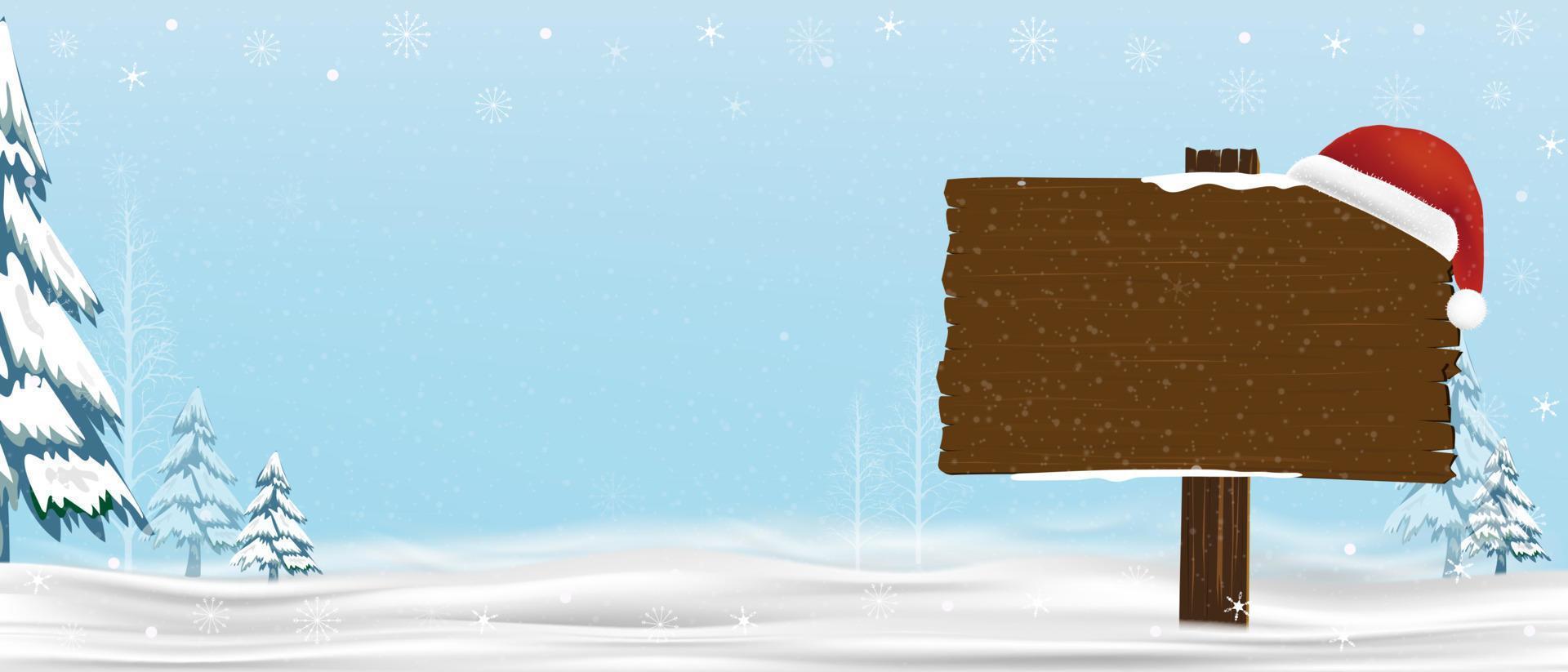The illustration depicts a charming, cartoonish Christmas scene, set in a snowy, wintry landscape. The ground is blanketed with deep snow, and evergreen trees, heavily dusted with white, stand proudly in the background. A flurry of large snowflakes gently cascades from the blue sky above. In the foreground, a wooden signpost, partially covered in snow, stands with a classic red and white Santa hat - complete with a fluffy white puffball - playfully resting on its right corner. Though the sign is blank, the whimsical setting suggests it could easily be used for a festive message or as part of a cozy holiday scene, reminiscent of a screenshot from a Christmas-themed game or a heartfelt greeting card.